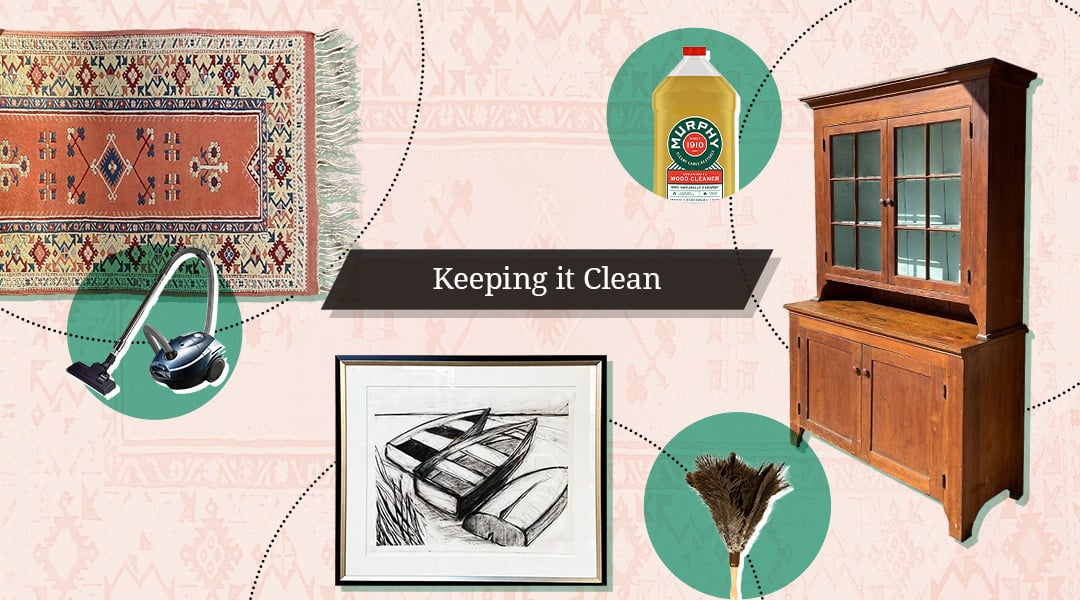This advertisement for Murphy's Oil Soap features a rendered, vintage-style image with various cleaning elements. Dominating the center, a bold black rectangle with white text proclaims "Keeping it Clean." Surrounding this slogan are several items showcasing the product's versatility. 

Towards the top left, there's a detailed burgundy oriental rug with intricate designs, indicating it can be cleaned with the product. Below it, a green circle contains an image of a vacuum cleaner, further emphasizing the theme of cleanliness. Centrally located at the top is another green circle displaying a bottle of Murphy's Oil Soap, the focal point of the ad. 

To the right of the bottle, a wooden hutch with glass doors and shelving illustrates one of the surfaces you can maintain with the oil soap. Directly beneath the black rectangle, there's a framed line drawing of rowboats, suggesting that even delicate items can be cleaned. Additionally, another green circle to the right contains an image of a feather duster, implying versatility in cleaning tools.

The background of the image is a soft, pale pink with a subtle diamond texture, resembling the design of a faded oriental rug, which complements the overall vintage aesthetic of the advertisement.